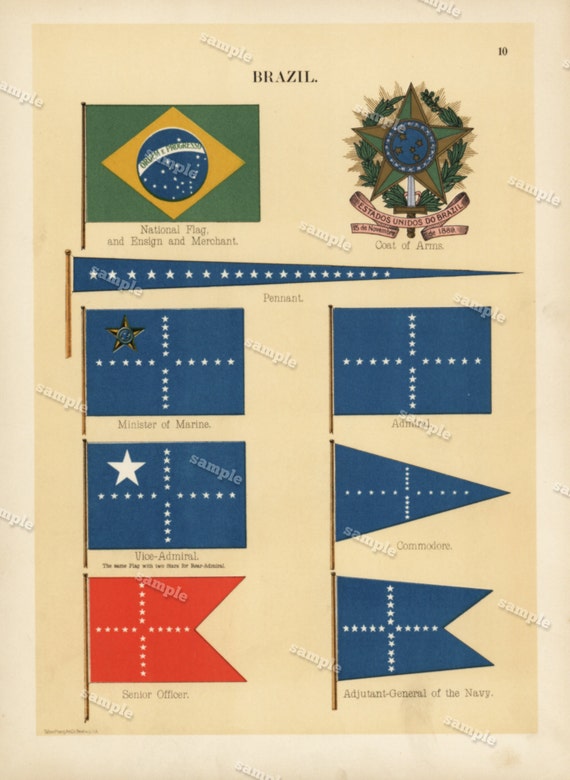This is an image of what appears to be an 8 by 10 piece of beige paper, seemingly ripped out of a textbook, as suggested by the rough edges and the numerical "10" in the top right corner, indicating it might have been page 10 of a book. At the top of the page, the word "Brazil" is prominently displayed. Below this title is the Brazilian national flag, which includes the phrase "Ordem e Progresso" on a green background with a yellow diamond and a blue globe in the center. Next to the flag is the Brazilian coat of arms, inscribed with "Estados Unidos do Brasil, 15 de Novembro de 1889" in Portuguese. 

Underneath the national symbols, there are several flags representing different ranks or roles within Brazil's military hierarchy. These include: a flag for the "Minister of Marine," which is a blue square flag featuring a T-shaped pattern of white stars with one prominent gold star in the top left, a red flag with a similar T-shaped pattern of white stars designated for a "Senior Officer," a triangular blue pennant, and a red rectangular flag for lower-ranking positions. Additionally, some flags specifically label roles such as "Vice Admiral" and "Adjutant General of the Navy," each distinct in color and star pattern.

The entire document is marked with the word "SAMPLE" across it, indicating it is a sample photo, likely used for illustrative purposes in educational materials. The intricate details of the flags and their distinctive patterns suggest their importance in denoting rank and authority within Brazil's naval and military services.